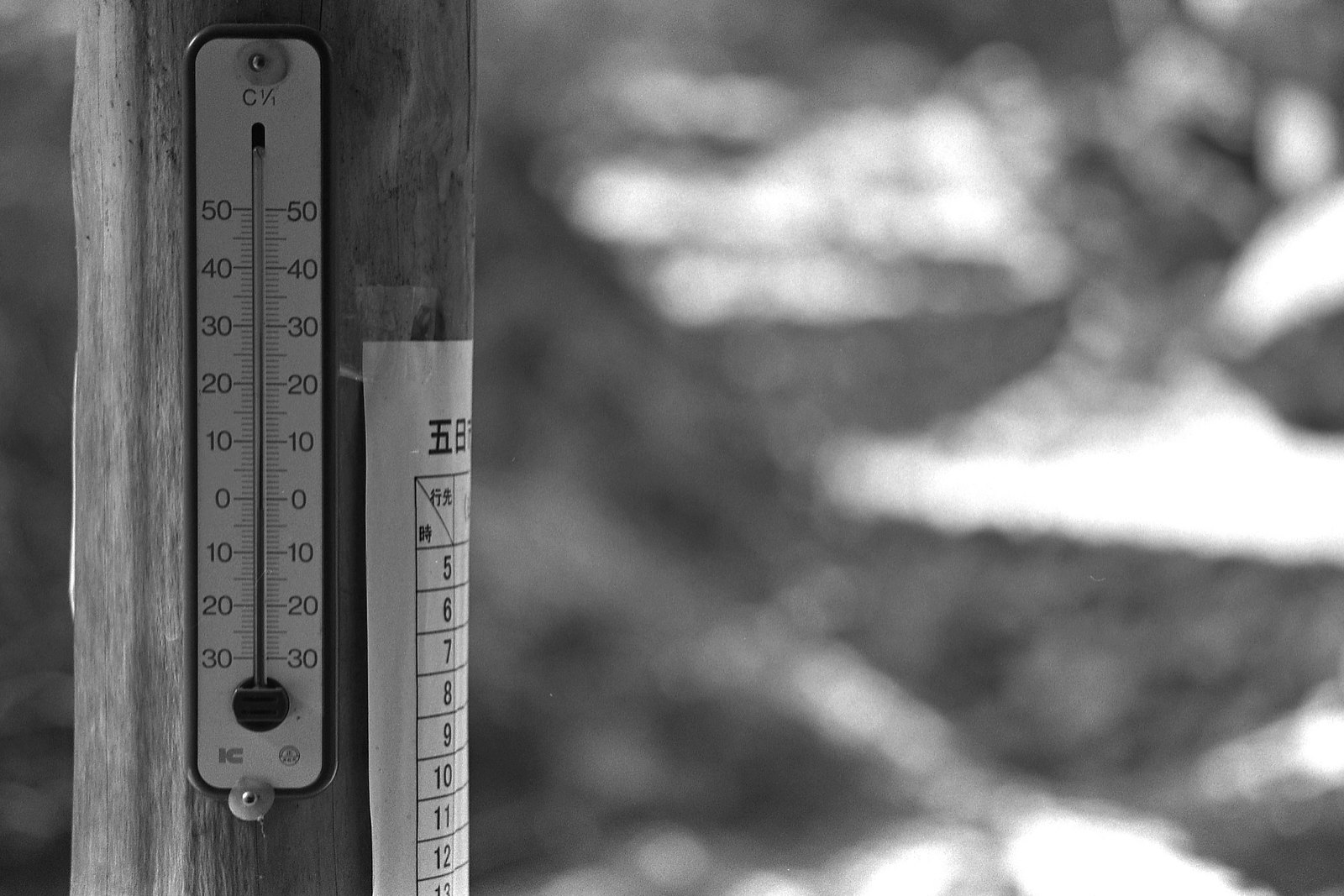In this black-and-white outdoor photograph, a prominent wooden pole is pictured on the left side, featuring a white thermometer attached to it. The thermometer, displaying temperatures predominantly in Celsius, has a range that starts from -30°C at the bottom, increasing through intervals of 10 degrees, reaching up to 50°C at the top. This thermometer also has a dark-colored border framing it. Adjacent to the thermometer, a piece of paper is visibly taped to the pole, which is distinctly characterized by its vertical and horizontal grain lines, indicative of its wooden material. The background is blurred and filled with light, presenting a mixture of light gray, dark gray, and white hues, partially obscuring the view of what seems to be trees or bushes. Additionally, there are vague triangular shapes noticeable in the upper right-hand corner, adding an element of intrigue to the scene.